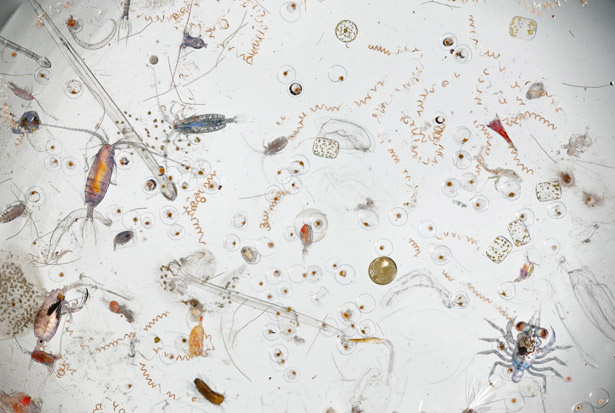The image presents an abstract, hand-drawn depiction of various bugs on a clean, white background. These bugs, or possibly microscopic creatures, are scattered throughout the image, each uniquely detailed. On the left, there's a purple bug with an orange center and long antennae. Above it, a smaller, compact bug with a blue center and grayish hue is noticeable. In the lower right, a creature resembling a spider has blue and gray legs extending outward. The background is filled with abstract designs, including brown swirling or squiggly lines and numerous shapes that resemble eyeballs with brown centers. Interspersed among these bugs are random objects such as marbles and dice, adding to the chaotic yet intriguing composition. The colors are vivid, with prominent hues of white, yellow, red, blue, pink, black, and orange. The overall focus seems to be on bugs, but the randomness and variety of shapes and details make it a complex piece to decipher.